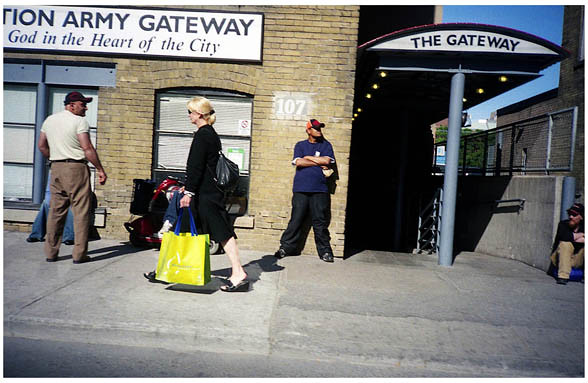In this color daylight photograph of a city street, we see a scene in front of a weathered light brown brick building that houses the Salvation Army Gateway, marked by a white sign that reads "Salvation Army Gateway: God in the Heart of the City." On the left side of the image, a man leans against the building with his arms crossed. He is wearing baggy black pants, dark shoes, and a blue shirt, complemented by an orange and black baseball cap. His gaze is directed to the left. Near the center of the image, a woman walks past, dressed in a dark outfit that appears to be either a skirt or long shorts and sandals. She carries a lime green bag with a blue strap in her left hand. In front of her stands another man, facing the building. He sports brown pants, a white t-shirt, and a dark baseball cap, looking to his right. The image also showcases a covered entryway with a sign that says "The Gateway" at the top, and in the background, another man in a black hat and top, with brown pants, sits against a concrete wall. The overall atmosphere is vibrant with sunlight illuminating the city sidewalk.